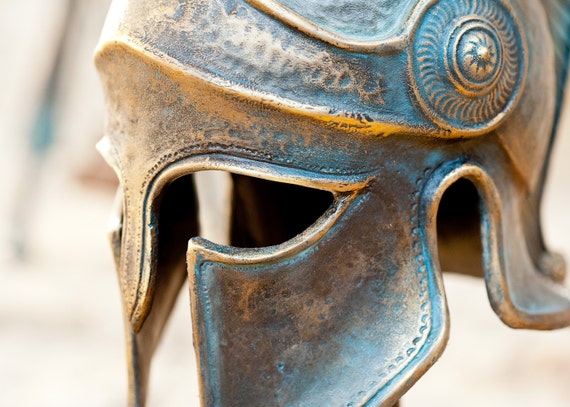This close-up photograph features a detailed and elegant ancient helmet, likely from a Greek or Roman military context, displayed against a blurred light brown-white background. The helmet itself is meticulously crafted from metal, exhibiting a yellowish-bronze color with areas of black, possibly showing signs of aging or wear. There are also hints of blue or green, suggesting copper elements or patina. Prominent above the ear on the left side is a circular design with internal lines and three smaller circles arranged in a pattern resembling a star. A defining stripe extends across the forehead and down the nose area. The eye openings are shaped in slits, providing a glimpse into the helmet's functional yet ornate design. This piece, with its graceful curves and intricate details, may be on display in a museum or similar setting, emphasizing its historical and artistic significance.